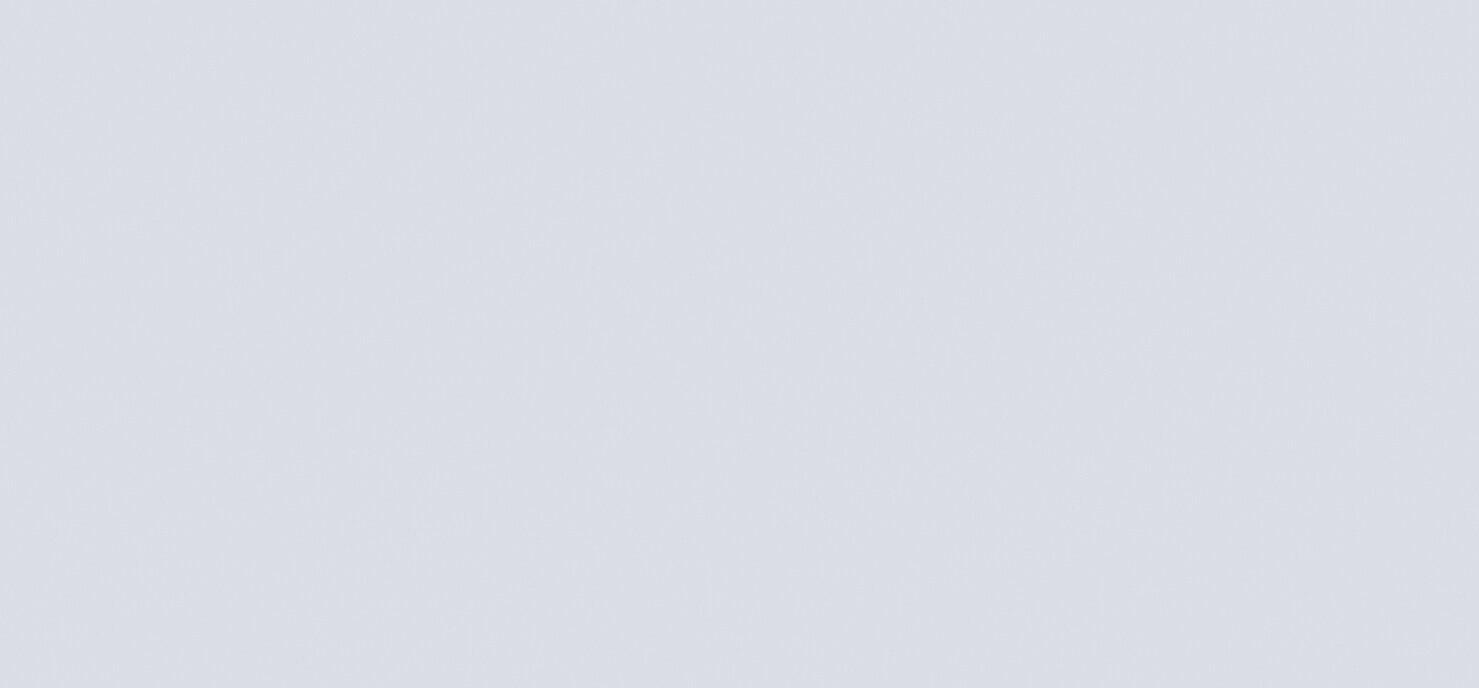The image features a medium gray, rectangular box centered against a plain white background. The box is oriented horizontally, spanning the entire width of the image. Measuring approximately three inches in height and eight inches in width, it has no distinguishing features or markings—neither graphics nor text. The minimalist composition draws complete focus to the plain yet sizable gray box, accentuating its simplicity and geometric form.